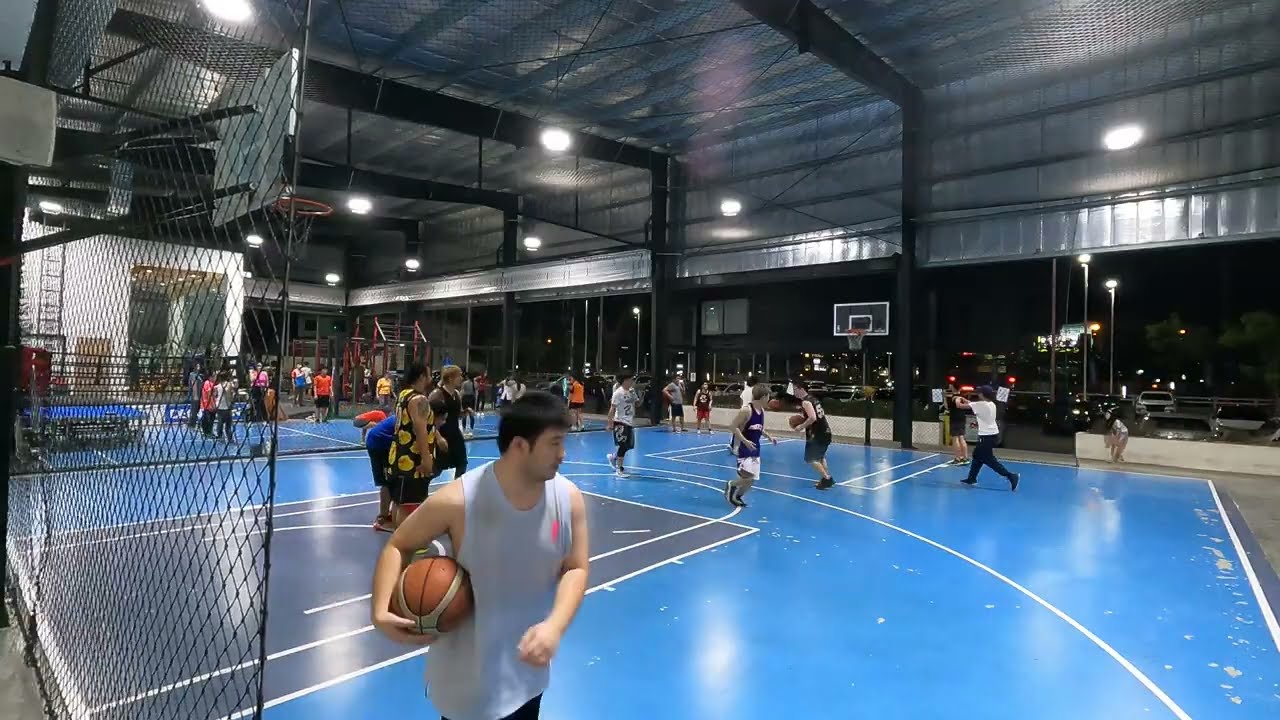This wide rectangular photograph captures the interior of a gymnasium, viewed from a corner on the short side of an indoor basketball court. The court's floor is a shiny blue material, with well-defined white and dark blue lines outlining the various areas of play. Several individuals, dressed in casual clothing, are actively engaged in drills, holding and shooting basketballs, indicating a practice session rather than a game. On the left side of the image, a black metal gate stands behind an orange basketball hoop with a white backboard. Adjacent to this court, another group of people can be seen, possibly engaging in gymnastics or another form of exercise, as they stand and move around. The top of the image reveals a tall, silver metal ceiling supported by black beams, with ample lighting illuminating the entire space. In the background, through what appears to be a transparent or open section, a parking lot with cars and street lights is faintly visible, suggesting the gym might be connected to or part of an outdoor covered area.